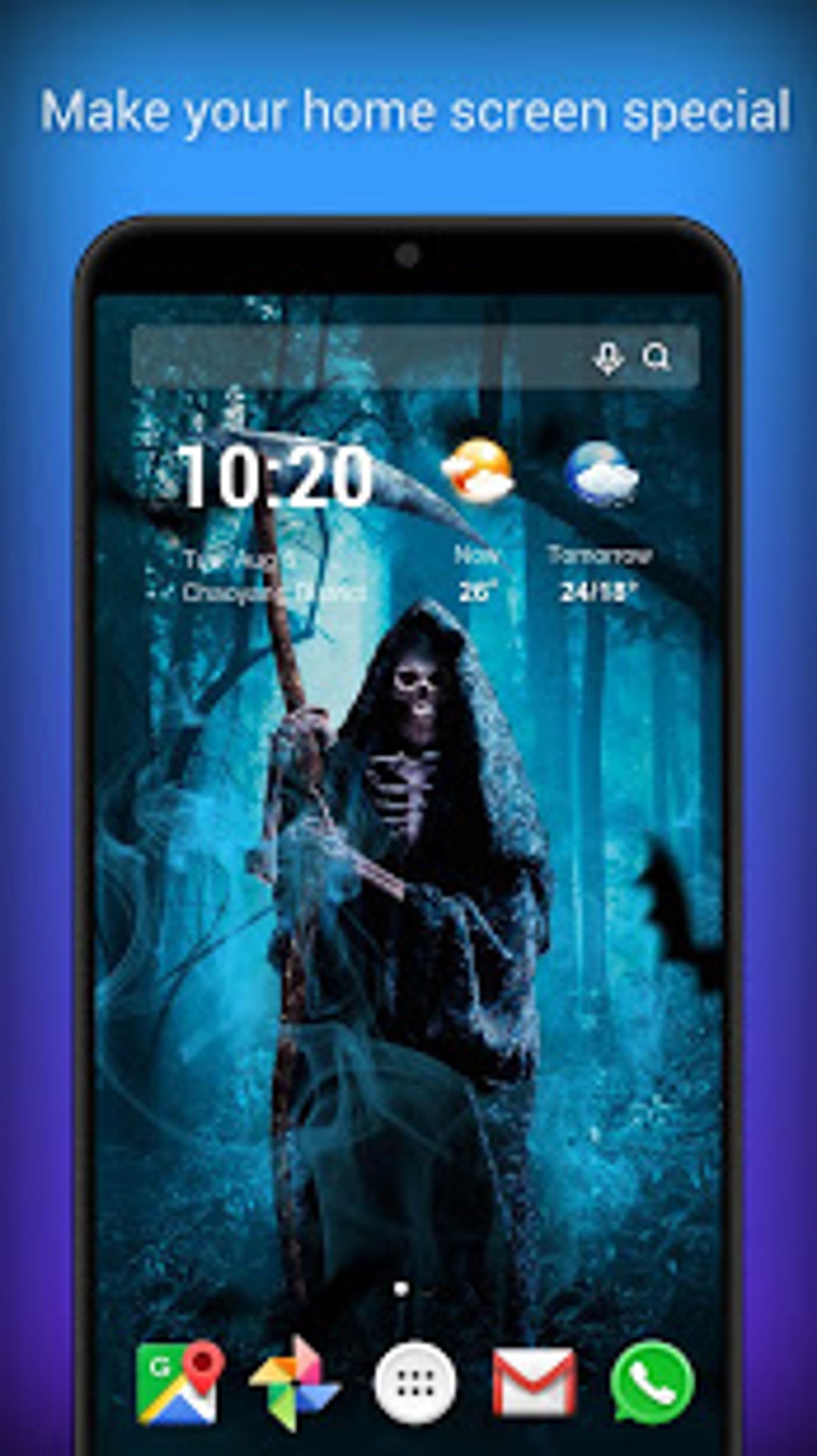The advertisement features a smartphone on an electric blue background with the text "Make Your Home Screen Special" prominently displayed in white at the top. At the center of the ad is a phone showing its lock screen, which has a Grim Reaper wallpaper. The Grim Reaper is depicted as a skeleton cloaked in a large, dark robe with oversized sleeves and a hood, holding a scythe. Surrounding the figure is a spooky nighttime forest with a teal blue tint, and a bat flies in the foreground. The time on the lock screen is 10:20, on a Tuesday, August 5th. At the top of the screen, there is a search bar, and beneath it, the weather information is displayed: "Now, 26°C" with a sun and clouds icon, and "Tomorrow, 24°C / 18°C" with a rain cloud icon. The bottom of the screen shows various Google app icons, including Google Maps, Gmail, and a button for all apps. The image has some blurriness, but the eerie details of the Grim Reaper wallpaper stand out.